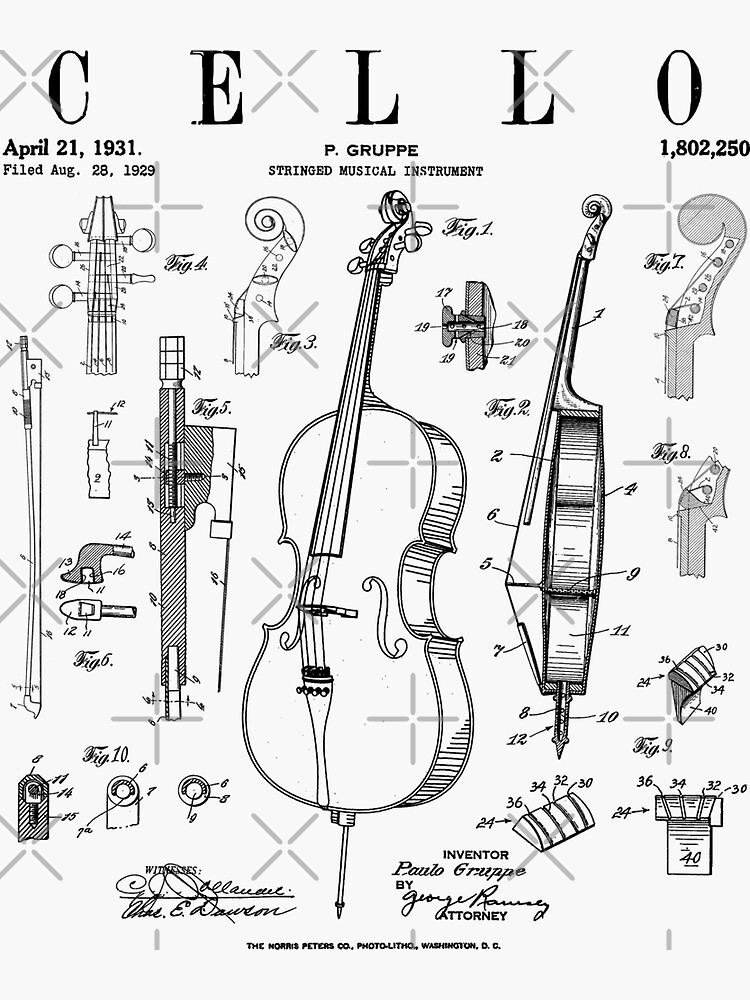This black and white diagram meticulously illustrates a cello with various detailed views and annotations. At the top of the document, "C-E-L-L-O" is prominently displayed, followed by "P. Gruppi, stringed musical instrument." Key dates are noted: April 21st, 1931, and filed on August 28th, 1929. On the far right, the patent number "1,802,250" is indicated. The main illustration of the cello is centrally placed against a white background, with a side view to the right. Surrounding these focal points are smaller, intricately labeled figures (Figure 1 through possibly Figure 10), mapping out specific parts of the cello with arrows and numeric references. Despite a lack of a specific legend for these numbers, the detailed figures provide a comprehensive breakdown of the instrument's components.